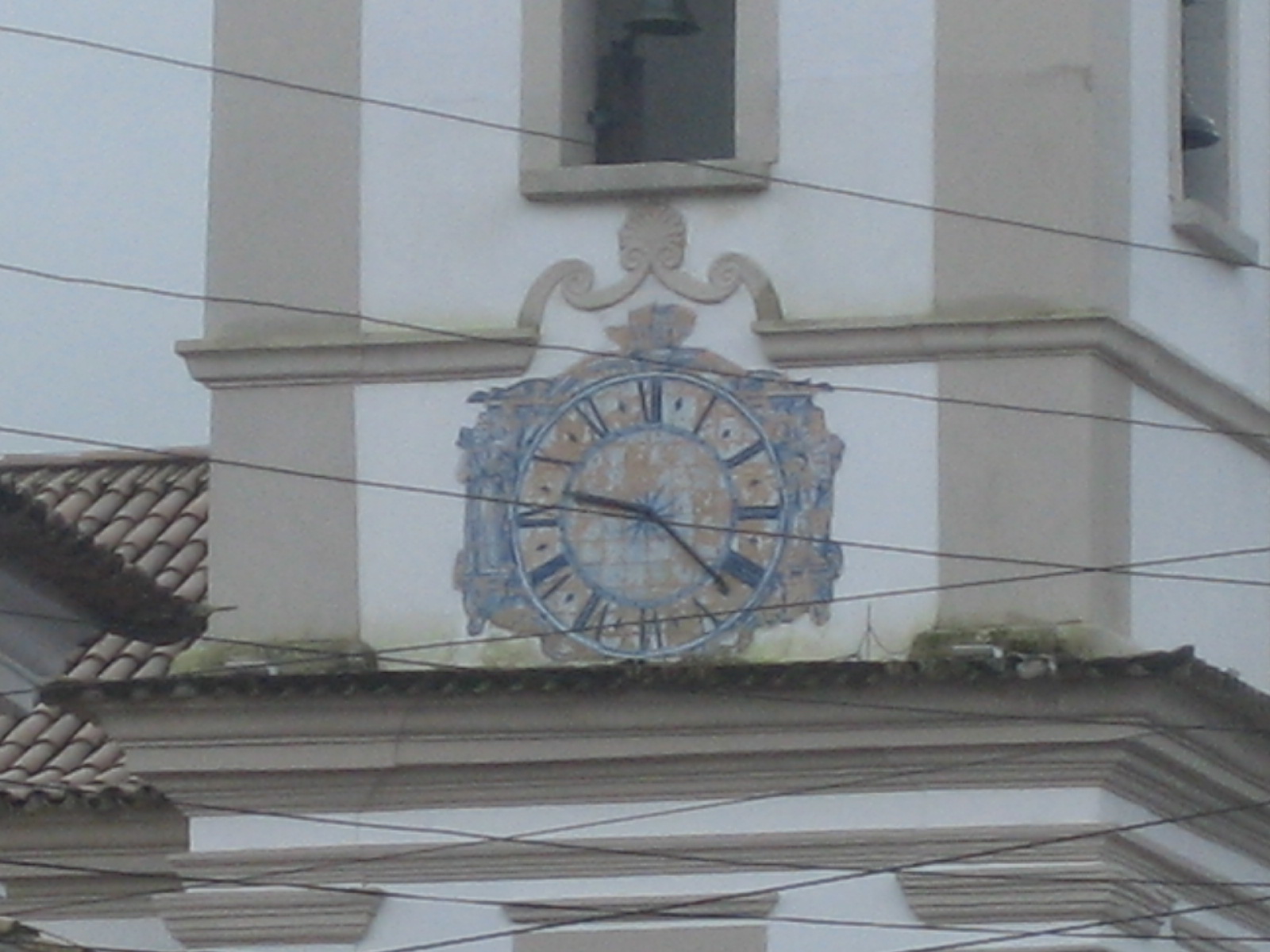This photograph depicts an intricately designed tower on a grand building featuring an elaborate clock. The clock face, which appears to be an analogue, prominently displays Roman numerals in bold black or dark blue, set against a backdrop of artistic orange-brown and brick-red tones. The minute and hour hands of the clock, rendered in brown, point to 22 minutes past nine. Surrounding the clock is a richly adorned, almost Asian-inspired architectural structure with gold outlines and decorations. Above the clock, a small bell is visible within a window bordered in brown, hinting at the tower's use as a bell tower. The building itself has a pale white and beige facade, accented by red-tiled roofs visible to the side. Horizontal power lines, numbering seven to eight, stretch across the scene, intersecting the view of the tower. This blend of detailed artistry and grand design creates a beautiful, complex visual.